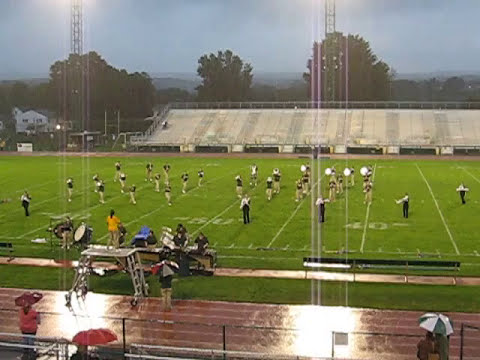The photograph showcases a high school football stadium during halftime, with a marching band in action. The green grass field features white football stripes and numbers, occupied by band members in khaki pants and black shirts, playing various instruments such as drums and tubas. A band leader, distinguishable by a yellow shirt, stands on a metal platform by the red running track that encircles the field. The track, with white lanes, appears wet, either from rain or the lights shining off its glossy surface. In the foreground, the image captures a few spectators underneath umbrellas, indicating the presence of rain, with a green and white umbrella visible at the bottom right corner. Flanking the bottom edge of the frame are the bleachers' first row and a railing. The background includes gray bleachers filled with more spectators, dark green trees, and towering metal light poles reaching into the overcast, darkening sky.